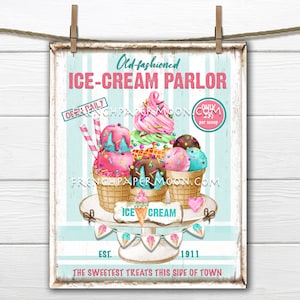The image features a nostalgic poster for an old-fashioned ice cream parlor, clipped with two wooden clothespins to a string against a white, wooden-slatted wall. The poster, which prominently highlights the phrase "Old-Fashioned Ice Cream Parlor" established in 1911, invites passersby to enjoy "the sweetest treats this side of town." The centerpiece of the poster showcases an array of colorful waffle cones filled with ice cream in vibrant shades of pink, blue, green, and chocolate, all topped with delicious sauces like strawberry and chocolate. Some cones also suggest swirled or soft-serve ice cream varieties, sitting temptingly atop a cake plate. The overall color scheme of the poster, featuring hues of white, turquoise, and pink, adds a charming vintage feel. Additionally, the poster bears a couple of faint watermarks.